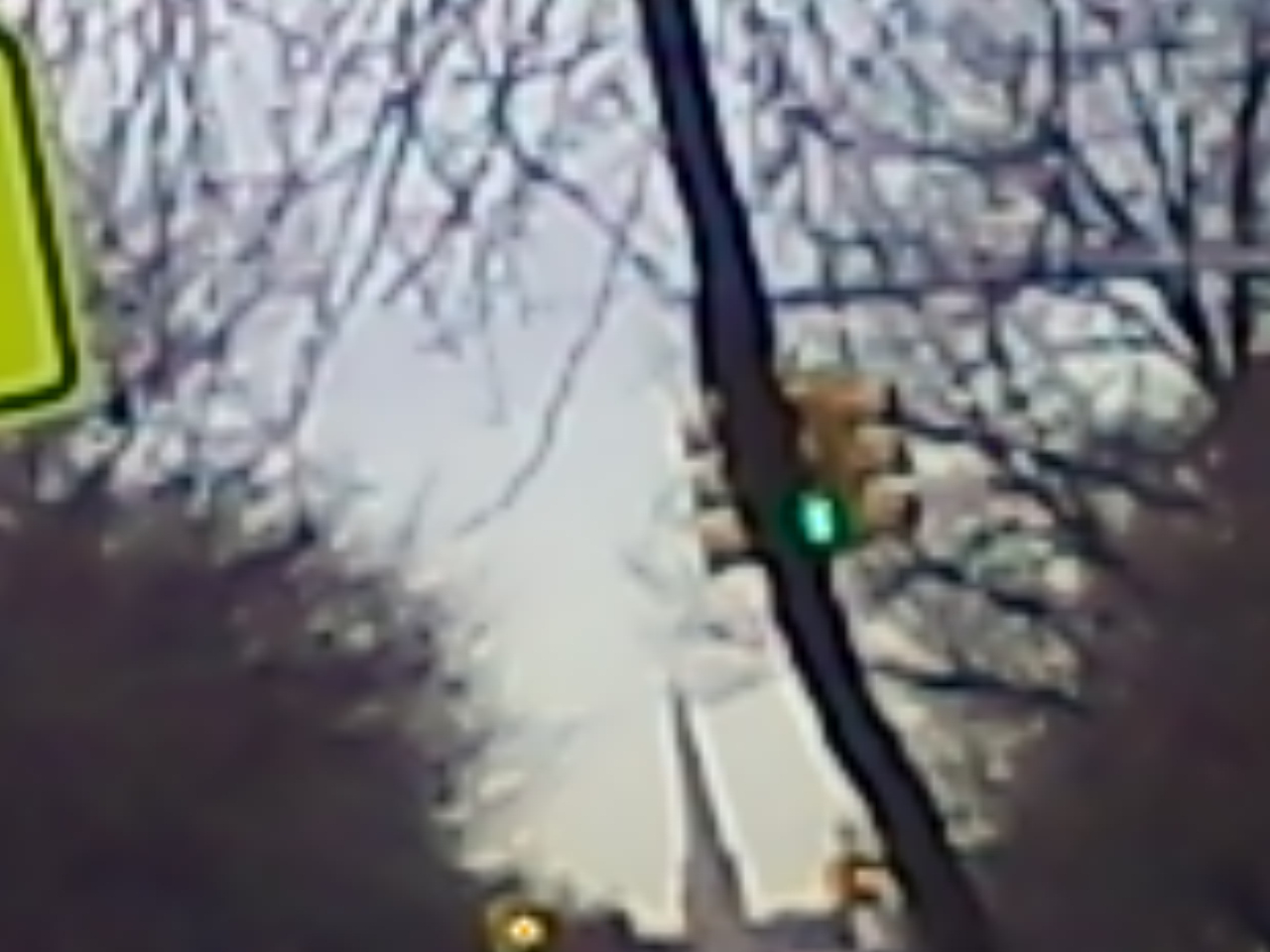This image, although extremely low in resolution and quite blurry, captures an outdoor scene, likely photographed using an older or obsolete device such as a phone or security camera. The focal point of the image is a traffic intersection where a single, beige-colored traffic light hangs suspended, swaying slightly in the wind with its green light faintly visible. The background reveals a wooded area with bare-branched trees stretching from the upper-left to the upper-right, suggesting it's taken during winter. To the left of the image, there's a partial view of a sign, outlined in yellow and trimmed in black, which could be a school sign. There's also an odd wobbly line crossing the image, possibly a tree branch or a screen artifact. In the distance, you can discern the faint outline of a church steeple rising up behind the trees. Overall, it appears to be a rural intersection captured perhaps from a security camera positioned to monitor the area, though no vehicles or pedestrians are visible.